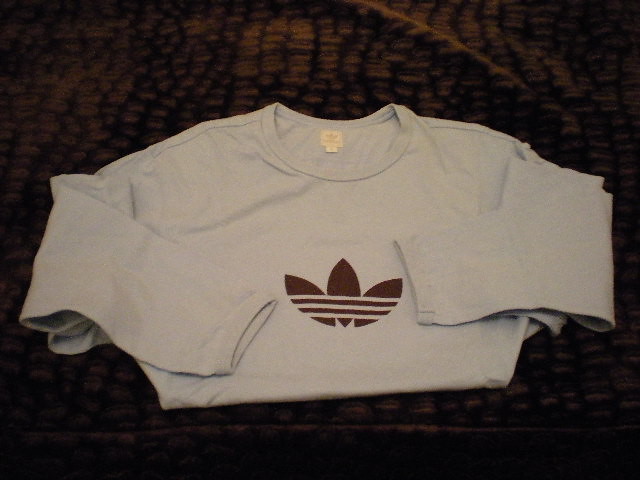The photograph features a horizontally long rectangular image. The background displays a snakeskin-like print in a combination of red and black colors, giving the impression of a textured fabric or blanket. On top of this background lies a folded white long-sleeve t-shirt. The t-shirt is neatly folded in half, with the sleeves tucked inwards towards the center of the shirt. Prominently displayed at the center of the t-shirt is the iconic Adidas logo, characterized by the three stripes extending across a trefoil design. An inner tag can be seen at the top center of the shirt, likely indicating the brand and size details. The collar of the t-shirt is a scoop neck featuring ribbed detailing that matches the white color of the shirt, as do the ribbed cuffs of the sleeves.